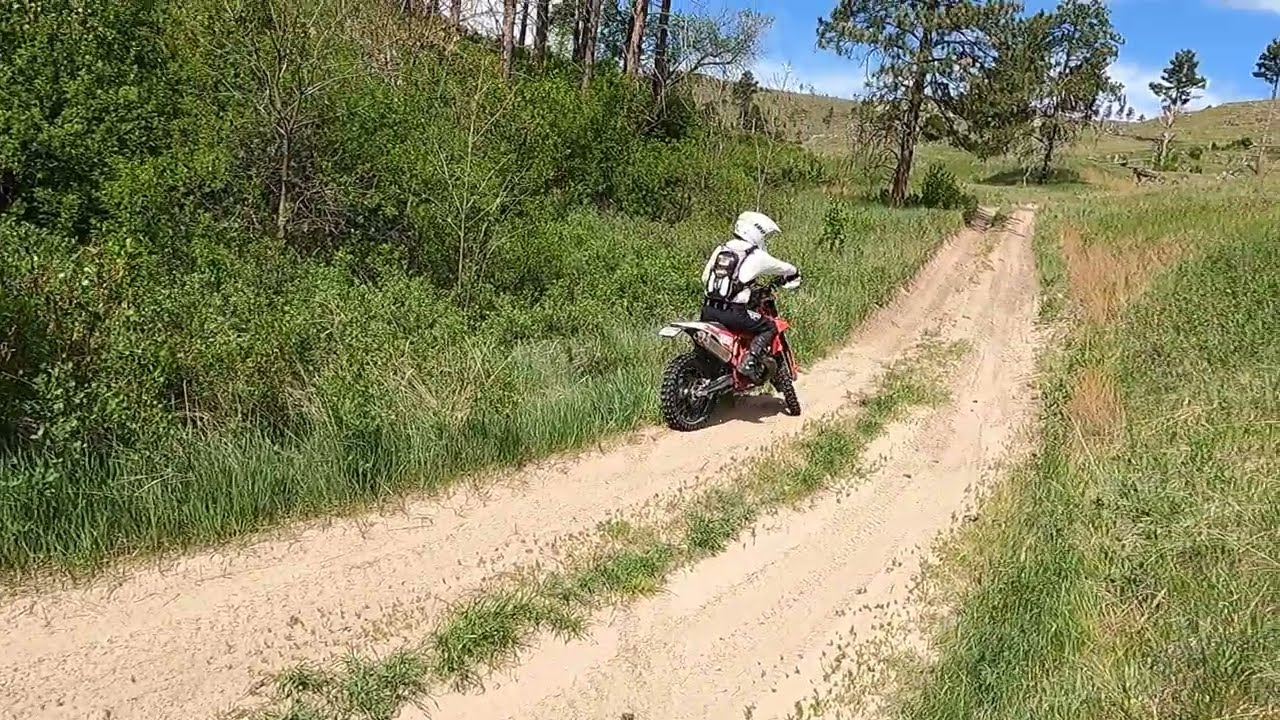The photo captures an off-road motorcyclist riding a red and white dirt bike along a dirt path on a partly cloudy day. The motorcyclist, equipped with a white helmet, white sweater, and black backpack, is facing away from the camera, with the front wheel of the bike slightly turned to the left. The dirt path is uneven and is likely created by tire treads, with rough grass dividing the trail. On the left side of the path, the terrain includes tall grass, shrubby plants, and a cluster of trees with visible trunks, ascending up a hill. To the right, the landscape features two trees with prominent leaves and is more open, sloping gently upwards with patches of dry grass. The scene is lit by the midday sun, highlighting the natural and rugged beauty of the area, while the scattered clouds add a dynamic element to the sky.